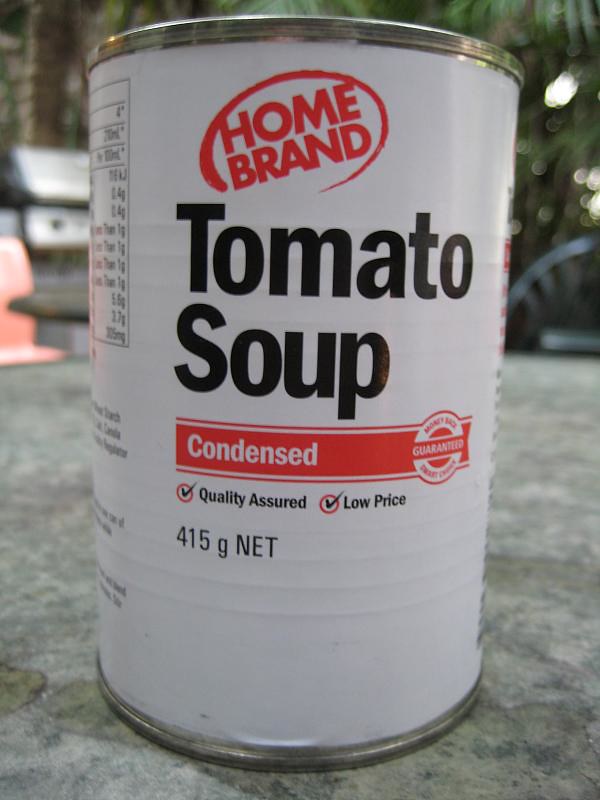This close-up color photograph captures a can of Home Brand Tomato Soup occupying almost the entire frame. The can features a silver rim at the top and bottom, with a white label showing slight greyish hues due to lighting. The label displays "HOME BRAND" in red letters within a red circle at the top. Below that, "TOMATO SOUP" is written in large black letters, followed by the word "Condensed" on a red band. Next to this, there's a red-and-white logo with the inscriptions "QUALITY ASSURED" and "LOW PRICE," each accompanied by a red circle with a black checkmark. At the bottom, the label reads "415 Grams Net" in black text. The side of the can reveals part of the nutritional information label, although it isn't fully legible.

The can rests on what appears to be a textured blue-grey or dusky green countertop, possibly laminate. The background displays a grey textured surface that could be either a table or the ground. In the top right corner, there are brown pillars, some foliage including trees, and light that illuminates a dark grey curved chair or possibly a gas grill, along with a hint of a red object or chair on the right-hand side. These elements suggest the setting might be a dining area, perhaps a restaurant with outdoor seating.